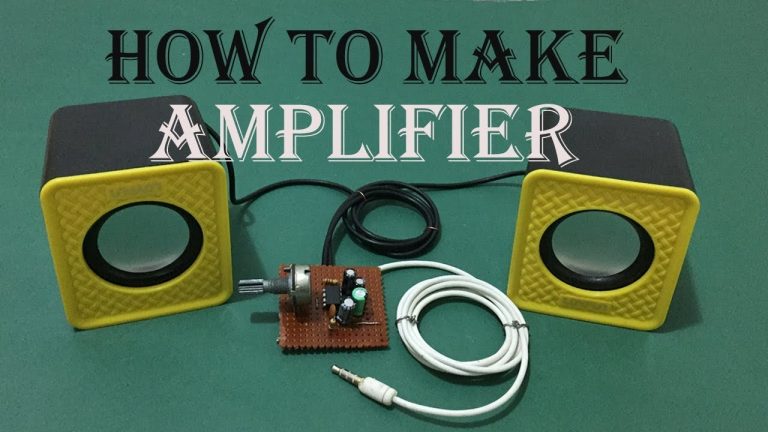The image features a green background with prominently displayed text at the top that reads "How to Make" in black letters, and "Amplifier" in white letters underneath. On the left and right sides of the image, there are two speaker-like devices with gray bodies and yellow front plates, each with a hole in the center resembling speaker cones. Extending from these speaker-like objects are black and white cords that connect to a central component resembling a control panel or motherboard. This central component is brown and populated with various electronic elements such as capacitors, chips, and a switch. Additionally, there's another white cord featuring what appears to be a headphone jack at its end. Overall, the setup is meant to illustrate the process of building an amplifier.